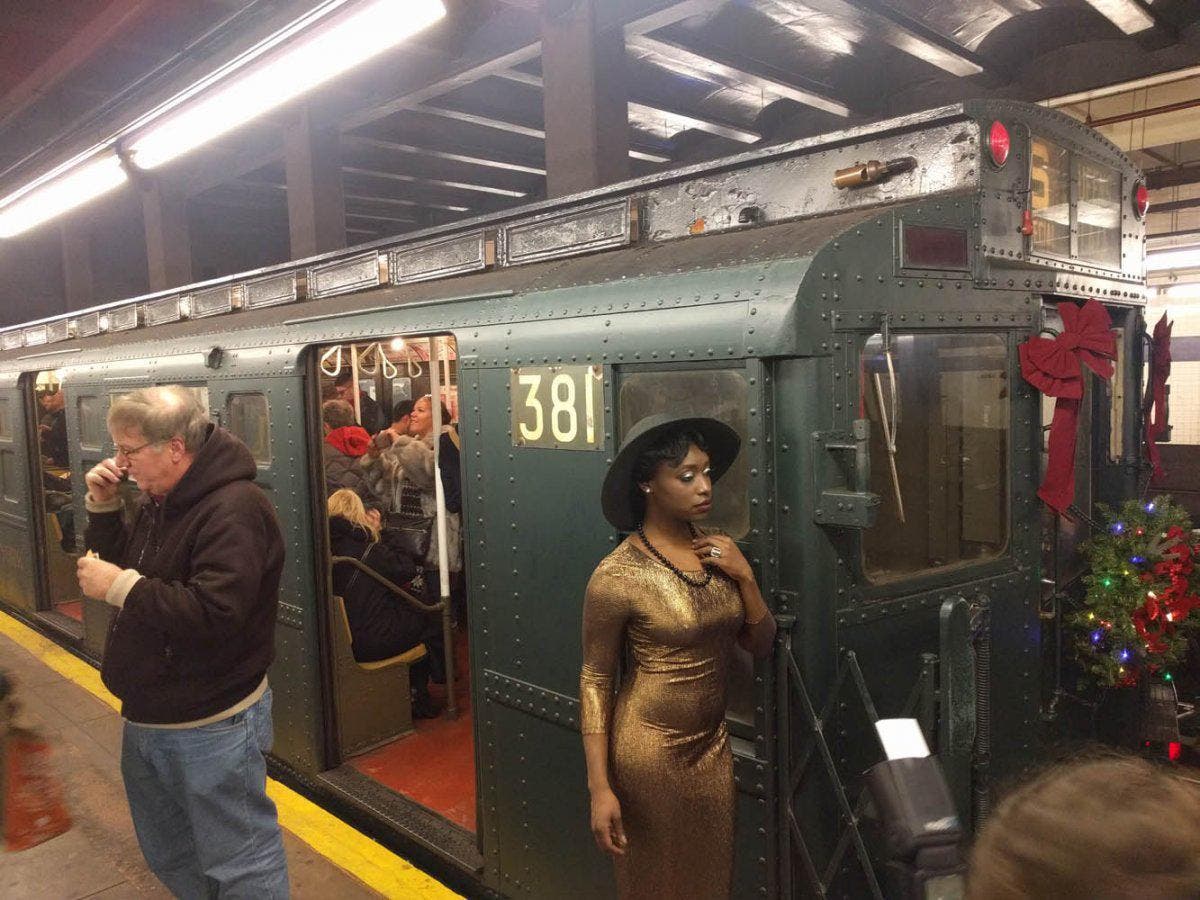The photograph captures a vibrant scene within an underground subway station, featuring an antique green subway car labeled 381. The car is adorned with festive holiday decorations, including red ribbons and a Christmas wreath with lights at the front. The interior hosts a crowd of people, both sitting and standing, depicted as non-distinct figures.

In the foreground, near the main entrance of the subway car, a black woman wearing a striking gold dress is captured walking away. To her left, towards the front, an elderly man dressed in modern attire of jeans and a sweatshirt is seen talking on the phone. Notably, there is also a woman with a black hat visible in the setting. On the bottom right corner of the image, part of a head is shown holding a professional camera, suggesting the picture was taken in a setting reminiscent of a museum, particularly one that captures the essence of urban transportation.

The overall scene likely takes place in a bustling city known for heavy subway use, such as New York City or Chicago, capturing a moment when passengers can board or alight the train.